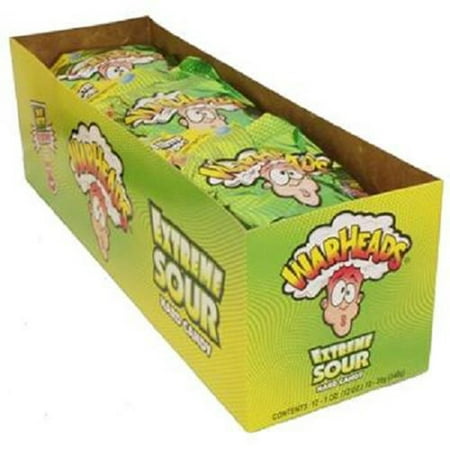This image features a slightly blurred, low-resolution photo of a lime green, rectangular prism-shaped box of Warheads Extreme Sour candy, positioned at a diagonal angle on a white background. The open top reveals three packages of the candy situated near the edge, implying that more packages are stacked below. The box and the candy packaging share a similar design, adorned with light green and wavy darker green lines. Prominently displayed on the box and packaging is a cartoonish white face with eyes bulging and lips puckering, signifying the extreme sourness of the candy. Above the character's head is a mushroom cloud bearing the word "Warheads" in gradient lettering that starts yellow and ends red. Underneath the face, the bold text reads "Extreme Sour" in green, repeated on the side of the box alongside the cloud-encased logo. Additional tiny text details the contents and weight of the candy but is too small to read clearly from the image.